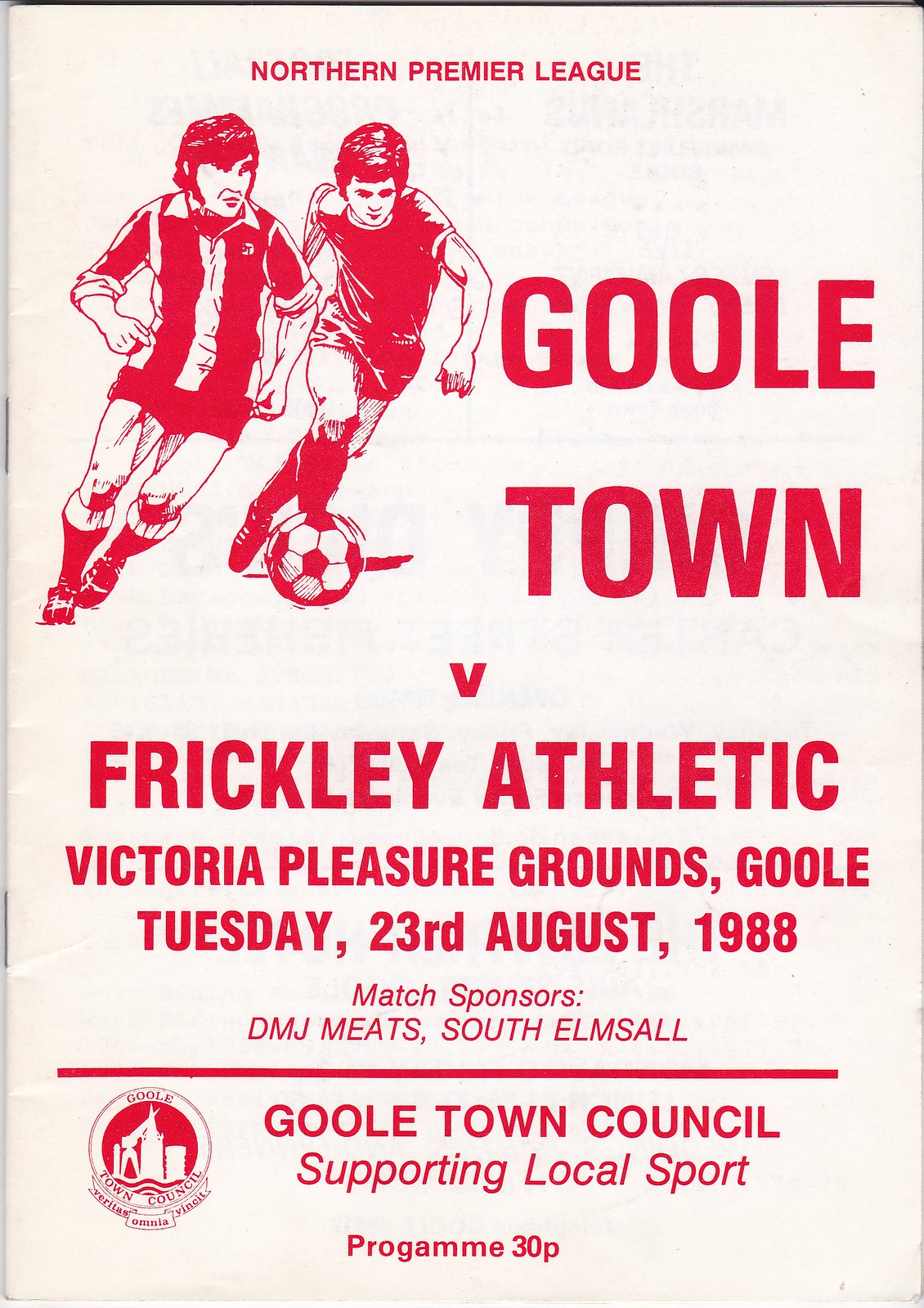This program flyer features a detailed, red-on-white design, commemorating a Northern Premier League soccer match. Centered at the top in small font, the text reads "Northern Premier League." Below this, a vintage, cartoon-style illustration captures two men in soccer uniforms mid-action: the player on the right is depicted with bent knees, poised to kick the ball with his right foot. To the right of the players, bold capital letters spell out "GOOLE TOWN," split across two lines, followed by "VS FRICKLEY ATHLETIC" in similarly prominent font. The flyer further details the venue and date: "Victoria Pleasure Grounds, Goole, Tuesday, 23rd August 1988." Lower on the page, in smaller text, it notes "Match Sponsors" with DMJ Meats of South Elmsall as a key supporter. At the bottom, the flyer highlights "Goole Town Council Supporting Local Sport," alongside the program's price of 30p and the town's emblem. The background sets a nostalgic tone with its aged, faint gray edging, indicative of its vintage 1988 origin.